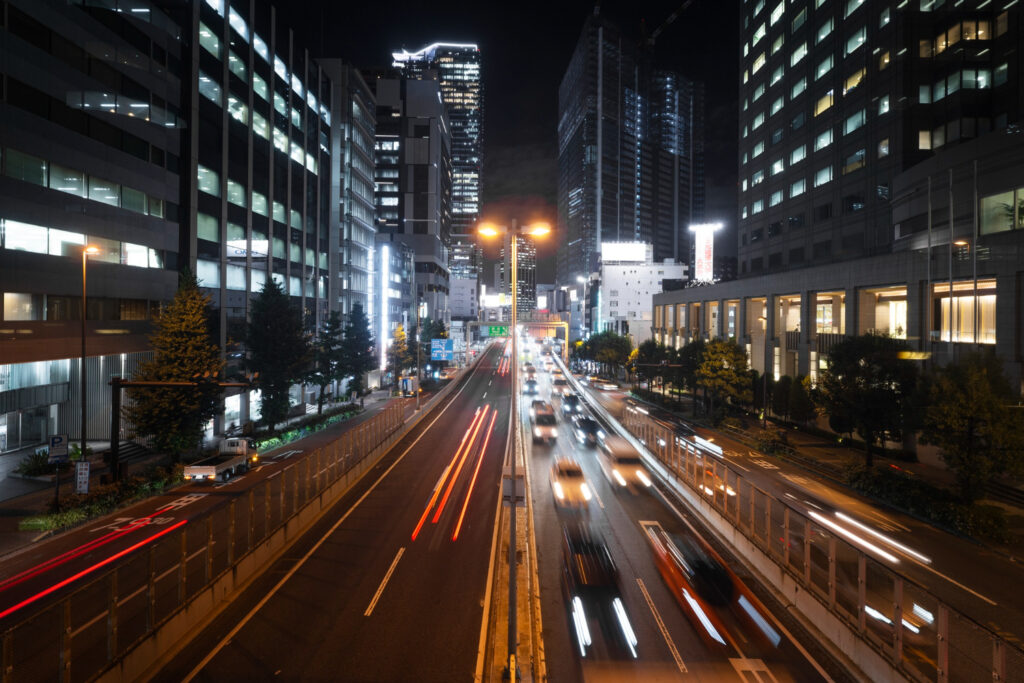This detailed photograph showcases a bustling city street at nighttime, capturing the vibrancy and motion through an artistic time-lapse effect. Set against a pitch-black sky, the scene is dominated by towering skyscrapers on both sides, their gray facades punctuated by numerous lit windows, which suggest office buildings or businesses. These high-rises stretch further into the background, getting taller and more distant, with one particularly tall building standing prominently to the right.

At the center of the image, a multi-lane highway runs through the city, with four lanes clearly visible—two in each direction—flanked by additional lanes on the sides. The traffic on this highway is a blur of motion, with elongated streaks of headlights and taillights creating a mesmerizing stream of light that emphasizes speed and movement. A white pole streetlight with two yellow lights on top is visible in the middle, contributing to the city's illumination.

Lining the sidewalks adjacent to the skyscrapers are small, neatly planted trees, and a handrail is visible, suggesting a pedestrian-friendly design. The city lights flood the entire scene with a warm, inviting glow, and some of the streetlights feature a prominent double-lamp design. The bustling energy and dense architecture, coupled with glimpses of Japanese writing on the road, hint that this could be a city in Japan, capturing a moment in the relentless flow of urban life.